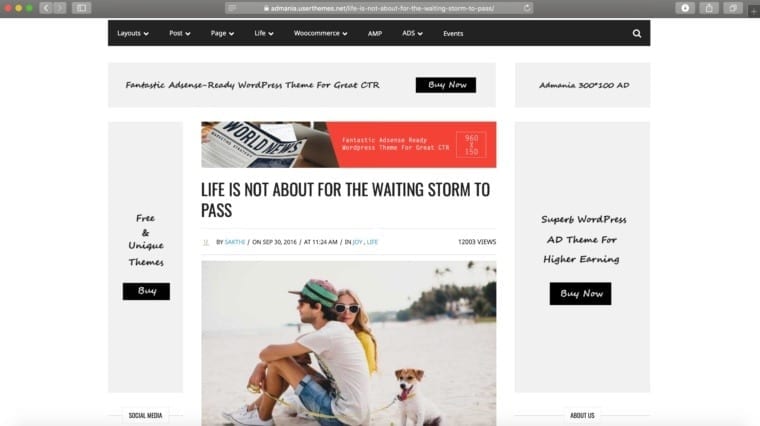This image appears to be a screenshot of a website viewed on a computer, though much of the detail is indistinct due to blur. At the top, there is a row of icon buttons, including a red dot, a yellow dot, a green dot, and arrows for navigating backward and forward. The URL in the address bar is not legible. Directly beneath is a black navigation bar with white text that is difficult to decipher. The first word might begin with 'L', followed by another possibly starting with 'P'. The words 'page', 'life', and a longer word starting with 'W' appear successively, each accompanied by a drop-down arrow. Further along, 'AMP' and 'ADS' (in capital letters) with drop-downs are visible, as well as what might be 'events'. A search icon is located on the right end of this bar.

Below this, a line of text, presumably reading "fantastic AdSense ready WordPress theme for great CTR," is partially legible but still blurry. There is a conspicuous "buy now" button underneath this text. Following that, there seems to be an advertisement, featuring a snippet of a newspaper headline that reads "world news." The ad includes a motivational phrase in capital letters: "LIFE IS NOT ABOUT WAITING FOR THE STORM TO PASS". Adjacent to this text is an image depicting a couple seated on a beach with a dog on a leash, enhancing the visual aspect of the ad.